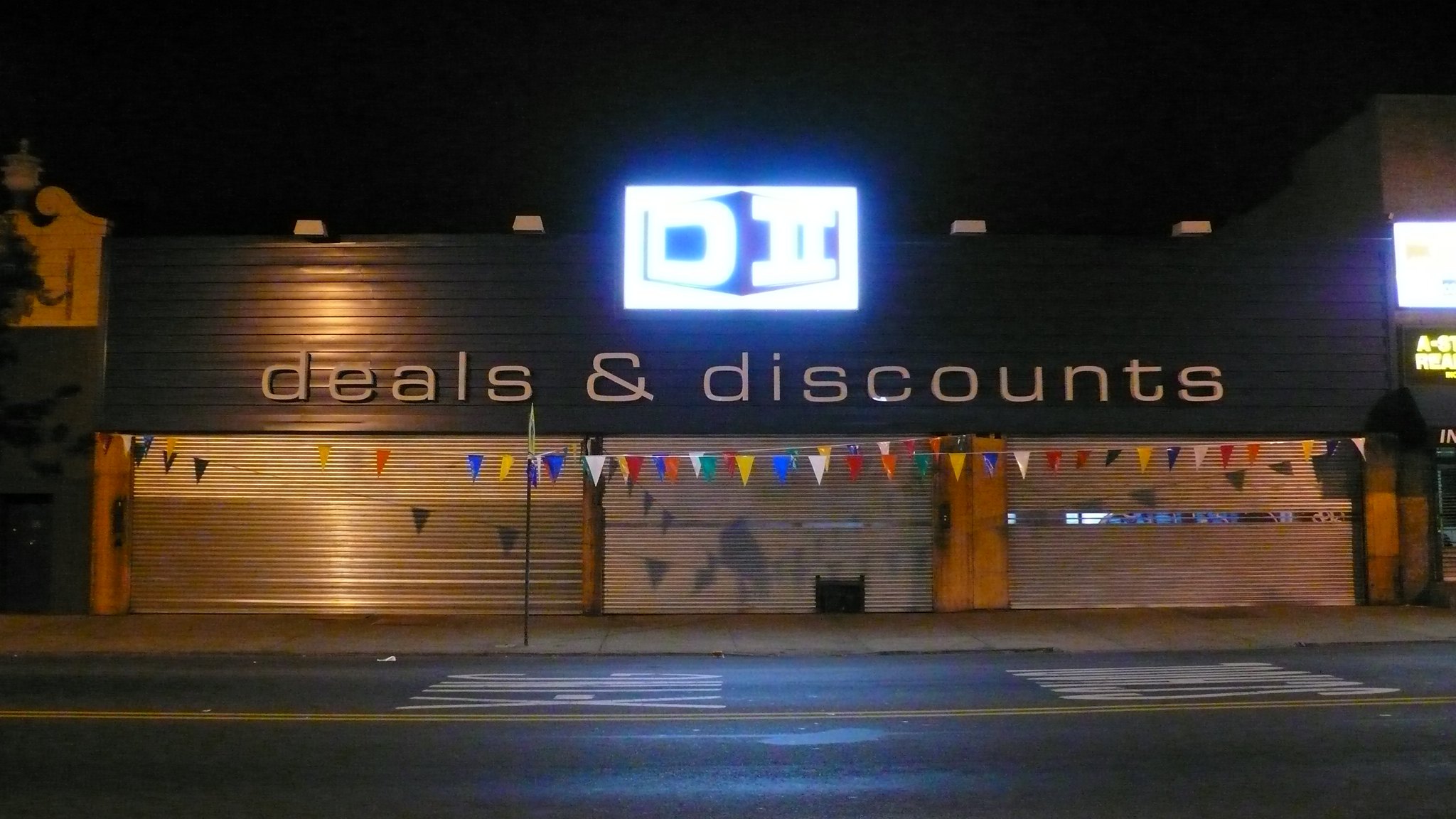The image showcases a long, rectangular building with a distinct appearance, suggestive of a repurposed structure such as an old mechanic's garage or a parking facility. The building's roof stands tall above the main structure, reminiscent of overhanging canopies, and is painted blue. Prominently displayed on the roof is the phrase "Deals and Discounts," written in bold white letters. The front façade of the building features three large, corrugated metal garage doors that further emphasize its industrial origin. Above the "Deals and Discounts" text, a neon blue sign captures attention with the inscription "D2," stylized within a rectangular frame. The letter 'D' is positioned on the left, while the Roman numeral 'II' appears on the right, both elements angling towards each other, creating a dynamic visual effect.